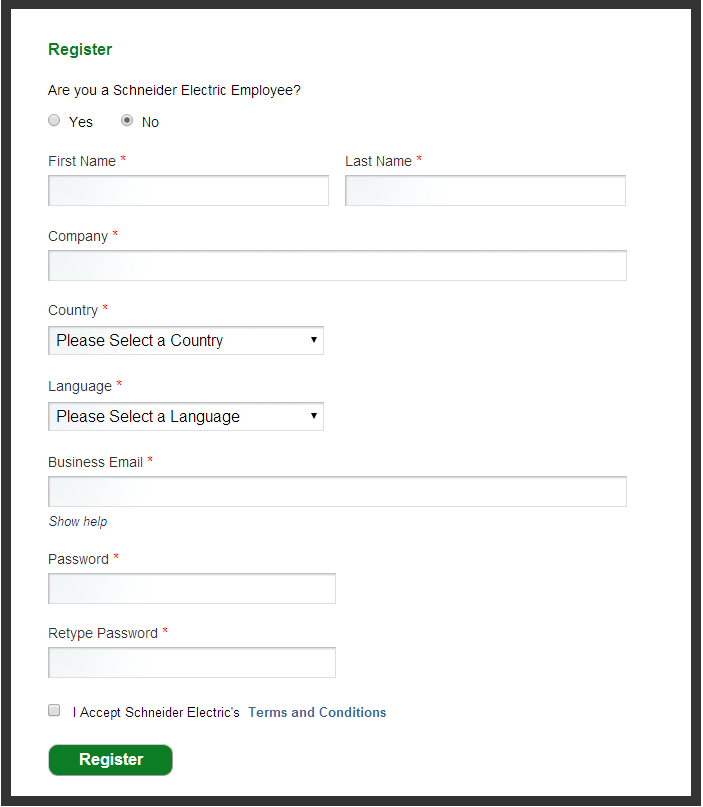The image is a screenshot of a registration form for Schneider Electric. The top section features the word "Register" prominently displayed in green text against a white background. Below the title, a question in smaller black text asks, "Are you a Schneider Electric employee?" accompanied by two buttons to select "Yes" or "No," with the default option set to "No."

The form is structured with multiple fields for user input:
- **First Name**: A text field on the left side.
- **Last Name**: A text field on the right side.
- **Company**: A field located beneath the first and last name inputs.
- **Country**: A dropdown menu for selecting a country, prefaced by the prompt, "Please select a country."

Following these fields is:
- **Language**: Another dropdown menu with the prompt, "Please select a language."

Further down, the form asks for:
- **Business Email**: Paired with a clickable "Show help" link in italics to offer additional guidance.
- **Password**: A field for creating a password.
- **Retype Password**: A field to confirm the password.

At the bottom of the form, there is a **checkbox** labeled "I accept Schneider Electric's terms and conditions," which is initially unchecked. The final element on the page is the **Register** button, intended to submit the filled-out form.

Overall, the screenshot captures a comprehensive and user-friendly registration process for gathering essential user information.